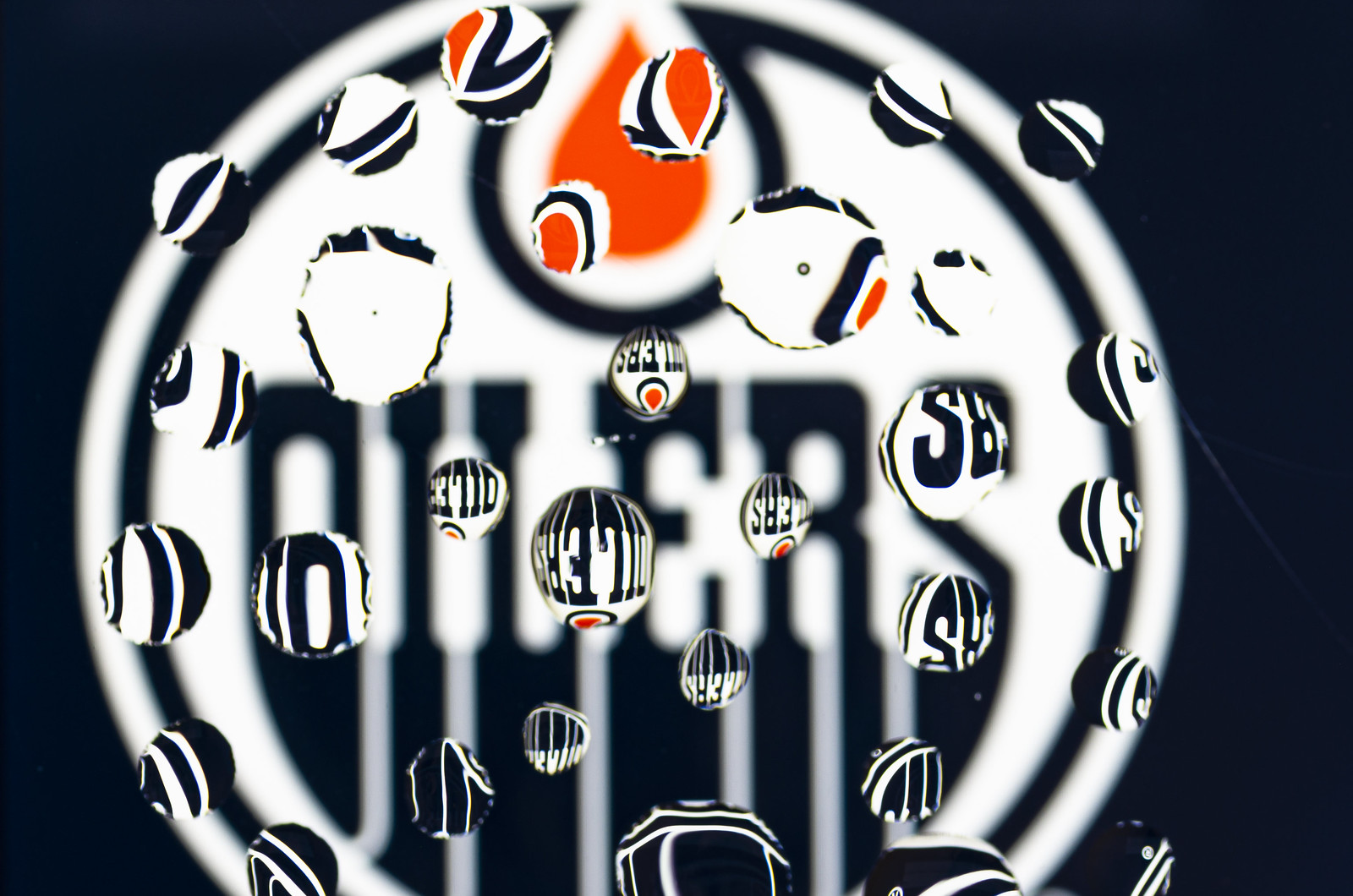This photograph captures an image of a round logo that prominently features the emblem of the Houston Oilers, though it should be noted that the Houston Oilers are an NFL team, not part of the NBA. The logo, possibly belonging to a company or another organization, displays a distinctive drop of oil atop it. The setup is dramatically backlit, enhancing the visual appeal of the scene. Overlaying the logo is a sheet of glass adorned with numerous water droplets. These droplets act as miniature lenses, refracting and inverting the logo within them. This intriguing optical effect results in a fascinating and unique image.